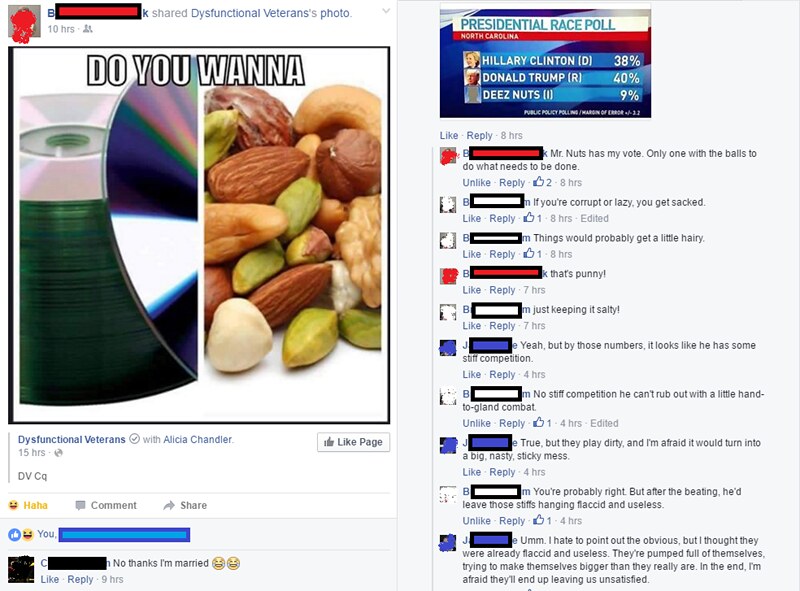The image is a dual screenshot from Facebook, featuring two different posts with humorous content. On the left side, there's a meme shared by a page called Dysfunctional Veterans. The meme displays a stack of CDs on the left and an assortment of nuts, such as peanuts and almonds, on the right, with the caption, "Do you wanna?" This is accompanied by Facebook reactions, including a "ha ha" reaction, with the original poster's name blacked out for privacy. A notable comment under the meme humorously responds, "No thanks, I'm married."

On the right side of the image, there's another post related to the 2016 presidential election. It shows a fake presidential poll from North Carolina featuring Hillary Clinton, Donald Trump, and a joke candidate named "Deez Nuts," who is humorously depicted with 9% of the vote. Trump leads with 40%, and Clinton has 38%. The post is followed by various comments that discuss the humorous nature of "Deez Nuts" as a candidate and make light-hearted jabs at the other candidates, particularly Trump. All names in the comments are blacked out for privacy.